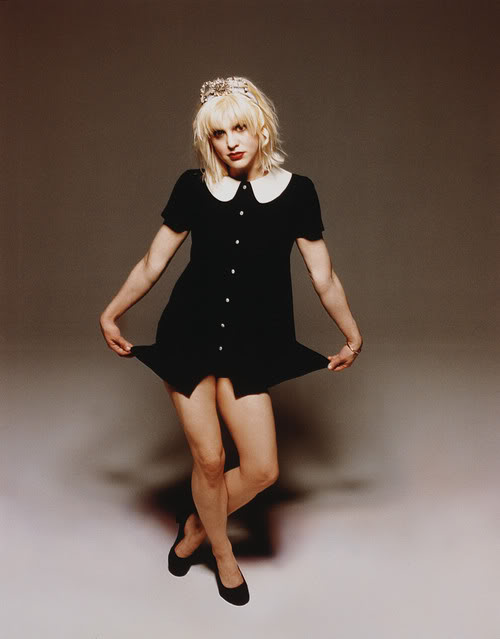The image depicts a professionally shot, vertically-oriented photograph of a woman who bears a striking resemblance to Courtney Love. She stands against a gradient background that transitions from dark brown to light brown. Her platinum blonde hair appears slightly disheveled and is adorned with a delicate tiara. She is dressed in a very short, black dress featuring a large white collar, short sleeves exposing her bare arms, and white buttons down the front. Completing her outfit, she wears black flat shoes and vibrant red lipstick. The woman is captured mid-curtsy, holding the edges of her skirt with both hands while crossing her legs and looking directly at the camera with a confident gaze. The backdrop includes shadows that add depth to the photograph, emphasizing her poised and elegant stance.